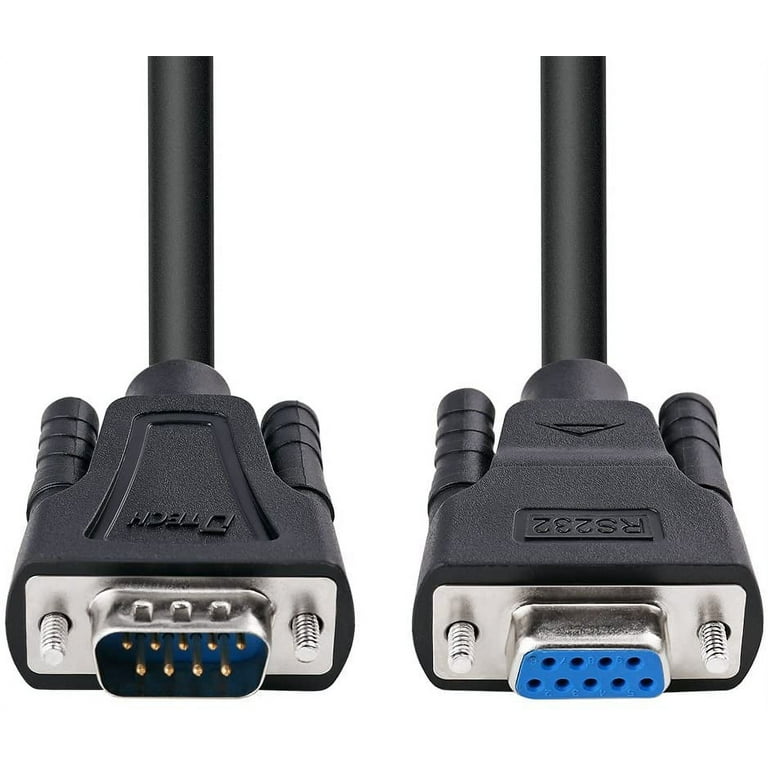The image showcases the ends of two black cables, commonly used for connecting older hardware to computers or televisions, displayed against a plain white background. The cables are constructed of black rubber and plastic with silver metal casings at the connecting ends. The left cable features nine gold prongs, encased in a protective silver sheath, with screws on either side for secure attachment. The right cable complements the left with nine corresponding holes designed to receive the prongs, also featuring screws for fastening. The right cable is marked with the text "RS232," while the left cable displays the partial text "GTECH." These connectors, identified as a male-to-female pair, ensure a secure and aligned connection, indicated by their matching screw mechanisms and alignment features.